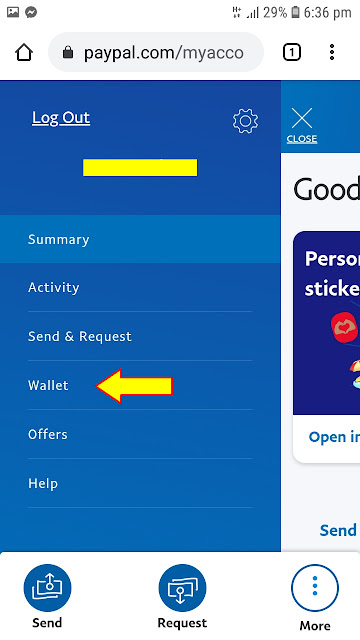The image displays a detailed user interface with various elements. At the top left, there is an icon featuring the familiar Instagram logo of the sun and mountain. Adjacent to it, a white speech bubble with a lightning bolt inside is prominently displayed. To the right of this area, white space dominates, and further to the right, there’s the text "H+" alongside an up arrow, a down arrow, and a "Full Self Service, 29%" indicator. A battery icon showing approximately 34% drain is also visible, along with the time stamp "6:36 PM."

The rightmost section of the top bar includes the outline of a house icon next to a grey bar partially overlaying the text "Paypal.com." Nearby sits a square marked with a number "1," indicating one open tab, followed by a three-dots menu icon.

Below this, on a dark blue background, "Blog Out" appears in white text on the left side, underlined to suggest it's clickable, with a gear icon on the right. Centrally placed beneath these elements is a yellow square digitally inserted, likely representing a placeholder for someone's name.

The interface transitions into a lighter blue and white section where "Summary" is listed on the left. It then shifts back to darker blue for options reading "Activity," "Send and Request," "Wallet," "Offers," and "Help." Notably, "Wallet" has an arrow pointing left directly beside it. On the far right, a lighter blue element has an underlined "Close" next to an "X."

Further down the page, a blue background reveals fragmented text, "PRSO" and "STIKE," hinting at some mention of stickers or possibly an incomplete phrase. The bottom section presents options to "Send," "Request," and "More," completing a complex but comprehensive user interface layout.